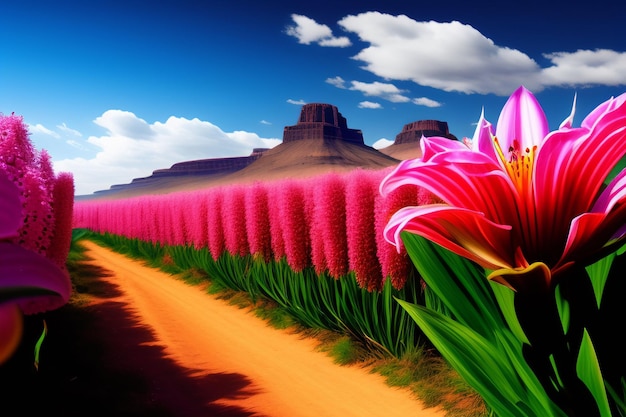This vibrant, computer-generated artwork, reminiscent of an oil painting, features a breathtaking southwestern landscape. Dominated by strikingly vibrant, hot pink flowers, the scene unfolds across a wide canvas. The flowers, almost resembling a fluffy corn maze, line both sides of a long, winding orangish dirt path that cuts diagonally from the bottom center to the left middle of the image. These tall, bushy flowers encompass the field, their brilliance accentuated by the lush green foliage at their base.

The sky transitions from a dark to light blue, dotted with a few clouds, suggesting a clear, warm day. In the foreground, to the bottom right, stands a single large hibiscus-like flower, distinct and grand compared to the other blossoms. This rich scene is set against a backdrop of majestic southwestern rock formations, akin to mesas or sand dunes. These formations support rustic, old-timey buildings, adding an element of historical depth to the piece. The painting-like quality and the meticulous detailing of each element make the landscape both enchanting and surreal.